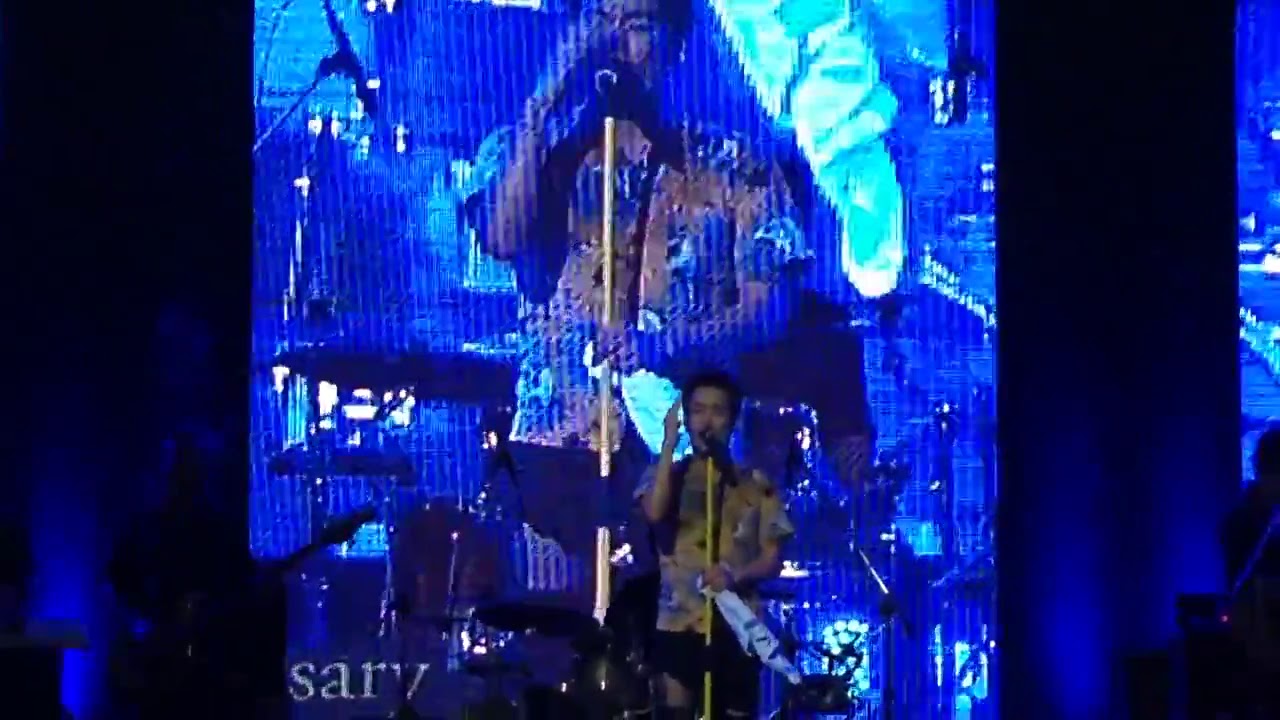The image captures a dynamic moment inside what appears to be a theater, filled with vibrant blue tones. The central figure is a young man, presumably of Asian descent, performing on a stage. He is wearing a short-sleeve, button-up Hawaiian shirt with tan and blue patterns, and dark pants. His left hand grips a microphone stand with a yellow mic, while his right hand is raised, pointing to his temple, emphasizing his performance. Behind him, a large digital screen displays an enlarged image of his face, zooming in on his expressive pose. Letters reading "SARV" are partially visible on the bottom-left corner of this screen. The backdrop of the stage is dark blue, adding to the dramatic ambiance. On the left side, there are balconies and possibly a piece of scenery crafted in blue, with a turquoise windsock-like structure hanging down with a white tip. The hints of musical instruments and a person with a guitar suggest that he is singing, fully immersed in the performance.